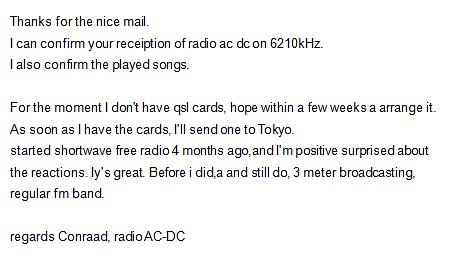This is a black and white, wide, rectangular image of an email with a completely white background and black, simple font. The email reads:

- "Thanks for the nice mail.
- I can confirm your reception of Radio ACDC on 6210KHZ.
- I also confirm the played songs.
- For the moment, I don't have QSL cards. Hope within a few weeks, I can arrange it.
- As soon as I have the cards, I'll send one to Tokyo.
- I started shortwave free radio four months ago and I'm positively surprised about the reactions.
- Before this, I did, and still do, three-meter broadcasting on the regular FM band.
- Regards, Conrad, Radio ACDC."